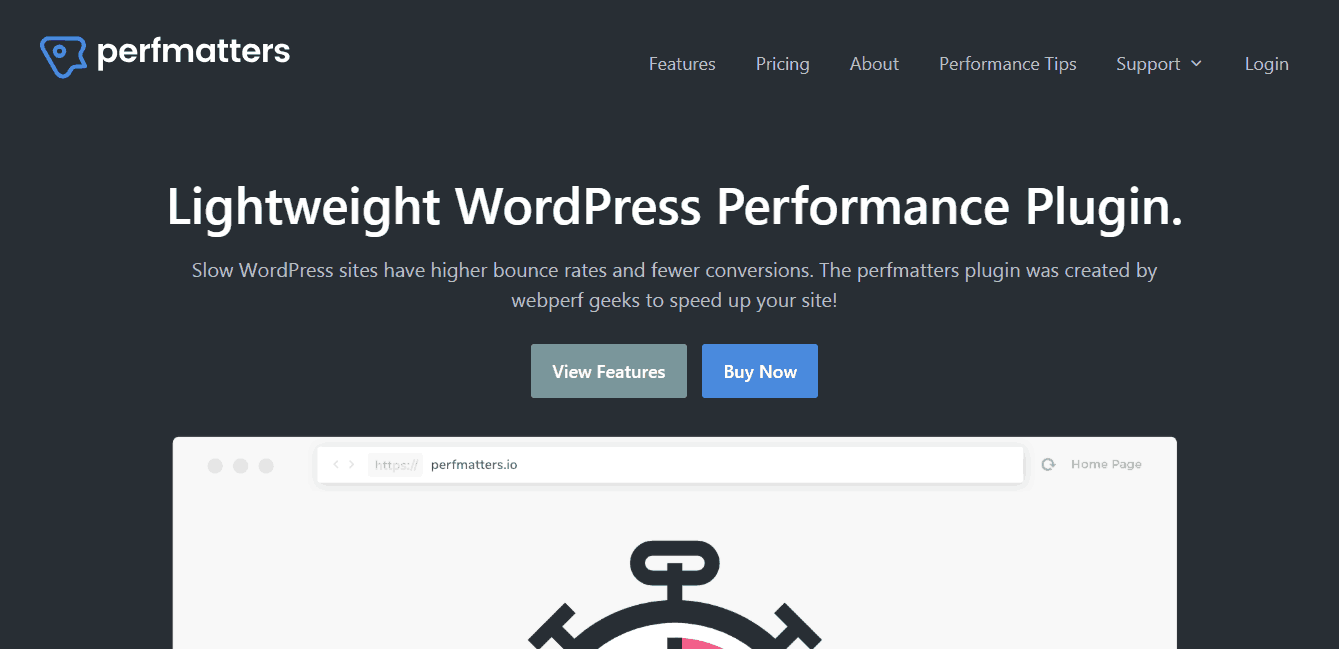The image showcases a web page from perfmatters.io, a website dedicated to a lightweight WordPress performance plugin designed by web performance experts. In the upper-left corner, there's a logo which seems to be a vector graphic, adjacent to the site's name, "Perfmatters," short for "Performance Matters." 

To the right of the logo, the navigation menu includes several items: Features, Pricing, About, Performance Tips, a Support dropdown menu, and a Login option. Below the navigation, a bold headline reads "Lightweight WordPress Performance Plugin," followed by the statement, "Slow WordPress sites have higher bounce rates and fewer conversions. The Perfmatters plugin was created by webperfgeeks to speed up your website."

The central part of the web page features a screenshot of perfmatters.io, showing the plugin's interface. Below the screenshot, there's an illustrated vector graphic resembling an irregular clock, with various decorative elements: a loop at the top, a vertical line connecting to the circular clock face, slanted lines at the 10 o'clock and 2 o'clock positions, each with perpendicular smaller lines on top, and color splashes of red-pink and black inside the clock face.

Two call-to-action buttons are prominently displayed beneath the graphic: "View Features" and "Buy Now."

Overall, the image represents a structured, professional layout of the Perfmatters website, emphasizing its core value of improving WordPress site performance.